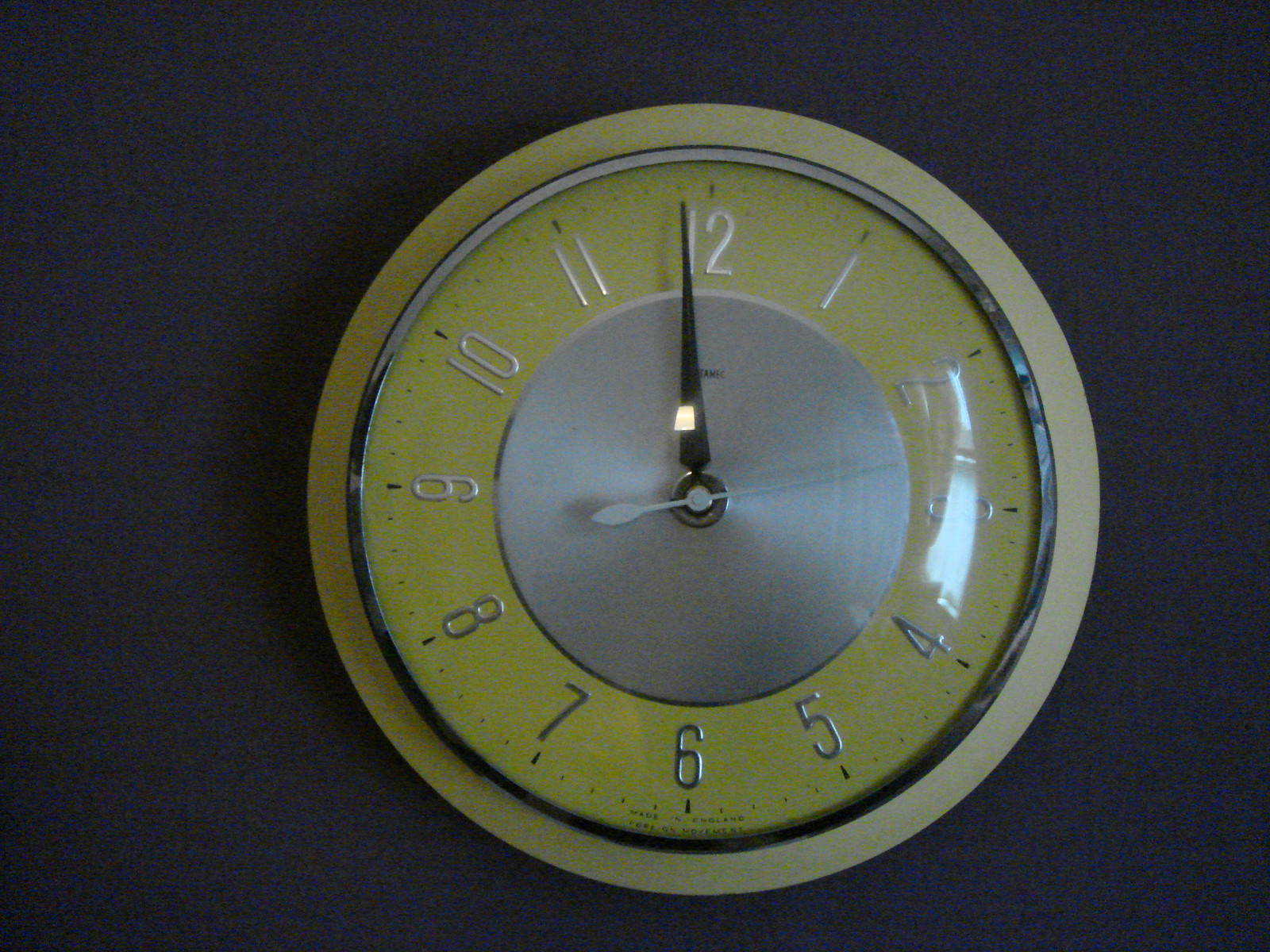This is a vintage-style wall clock, possibly from the 1950s or early 60s, against a dark gray or black background. The clock features a corkboard-like light brown outer ring, followed by a metallic silver interior. The section with the numbers is a buttercup yellow. The clock has silver Arabic numerals and black hour and minute hands, both almost pointing to the 12, indicating it’s nearly midnight or noon. The silver second hand is positioned between the 2 and 3. A reflective glass cover is attached to the yellow part, with a visible light reflection. A silver circle in the middle supports the hands. There is also an indiscernible brand name beneath the clock hands.